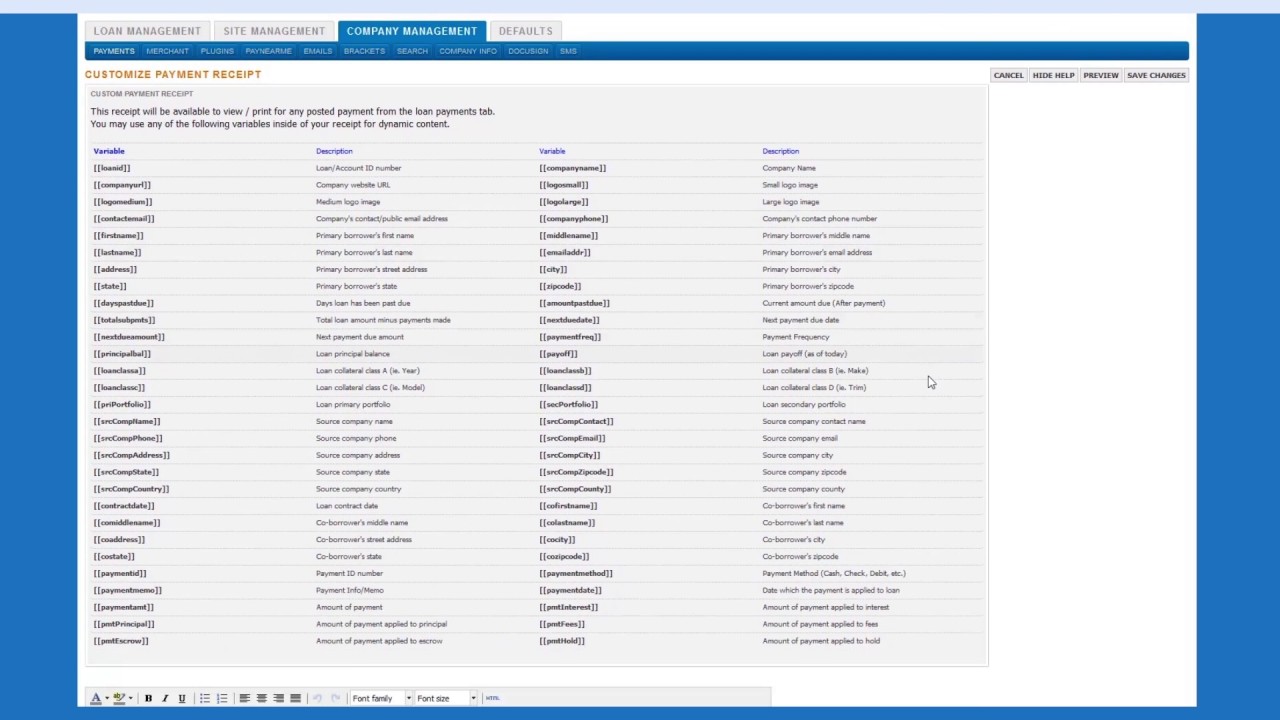The image displays a screenshot of a website interface designed for loan management. On the left side, a vertical blue line separates the main menu from the content area. The top of the menu features three main categories: "Loan Management," "Site Management," and "Company Management," with the "Company Management" tab highlighted in blue. Beneath this highlighted tab, a list of options is visible, including "Payments," "Merchant," "Plugins," "Pay Near Me," "Emails," "Brackets," "Search," "Company Info," "Docuzine," and "SMS."

The main content area is set against a white background. At the top, bold yellow text on the left reads "Customize Payment Receipt." Directly below, in black text, "Custom Payment Receipt" is displayed. The text explains that this receipt will be available for viewing and printing for any posted payment from the "Loan Payments" tab. Users are informed that they may use various variables within their receipts to include dynamic content.